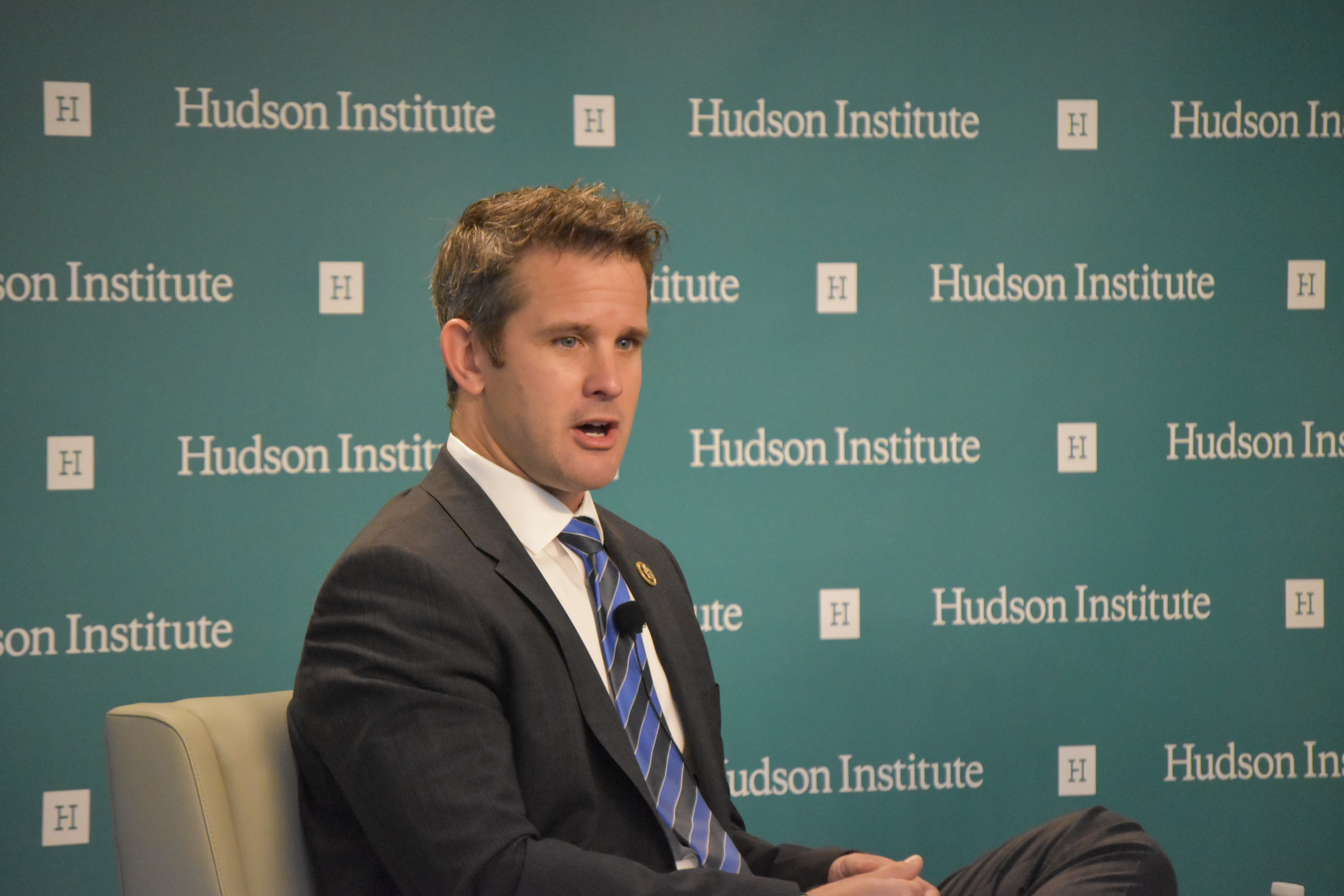The image is a detailed color photograph in landscape orientation, featuring the politician Adam Kinzinger. Kinzinger is seated in a tan-colored, leather-style chair with his legs crossed, and his knee is visibly poking from the bottom. He is looking towards the bottom right of the image at an audience that is out of view, with his mouth partially open, suggesting he is mid-speech. He is wearing a dark blazer, a white button-up shirt, and a blue and black striped tie. Attached to his tie is a round lapel microphone. The background features a dark teal wall banner adorned with the words "Hudson Institute" in white, repeated multiple times. Interspersed between the text are white squares with a green letter "H" in the center, arranged in horizontal rows. The photograph captures a moment of representational realism, emphasizing the formal tone and setting of the scene.